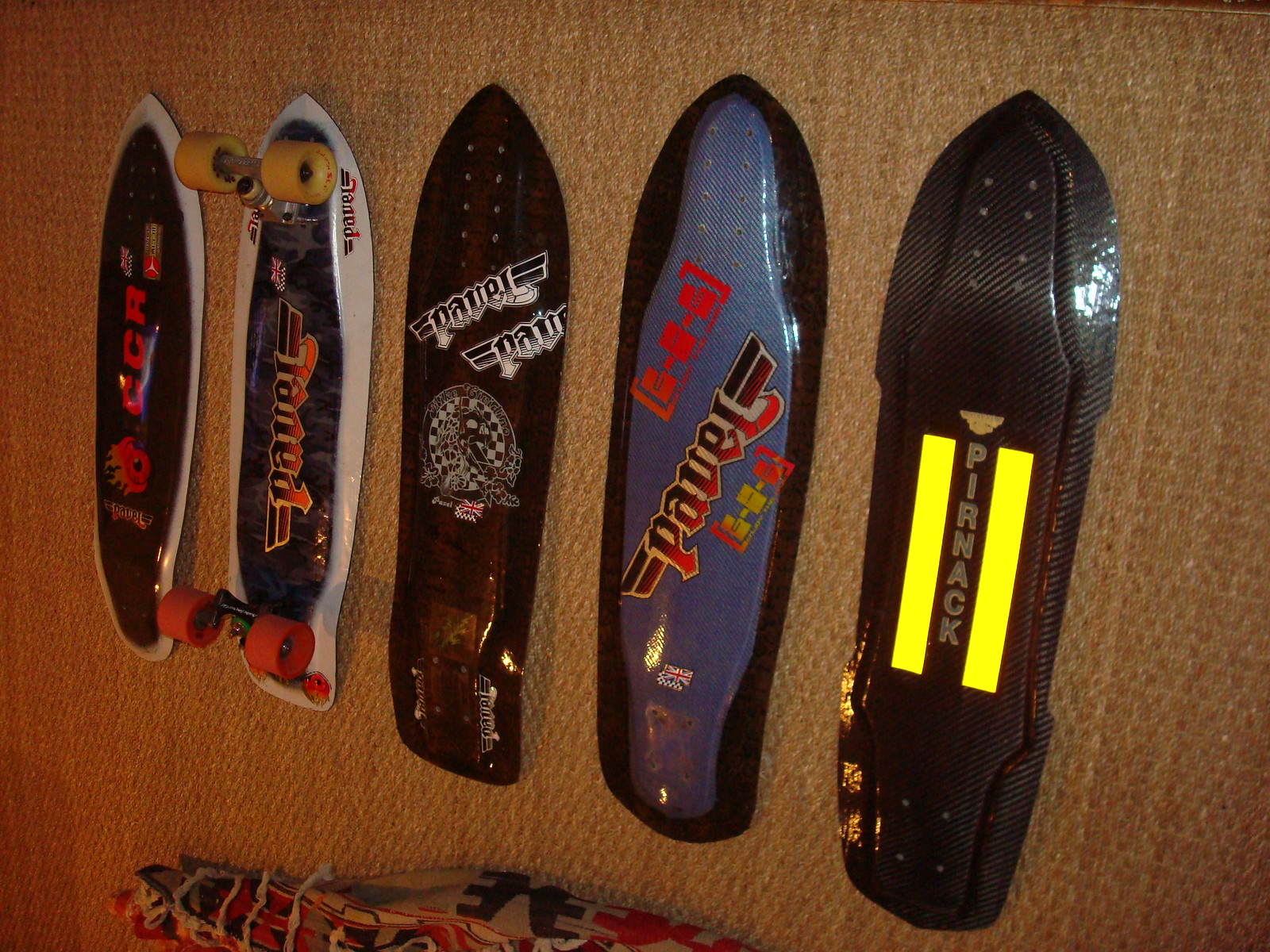The photograph captures five skateboard decks arranged vertically on a tan carpet. Four of the decks are without wheels, showcasing their unique designs, while the second board from the left still has its wheel setups intact, featuring light yellow wheels at the front and orange wheels at the rear. From left to right, the skateboards display distinct graphics and logos: the first deck is black with the letters "CCR" in red on a navy blue background bordered by white, the second deck is blue with a black outline and red, indecipherable text, the middle deck is black with a circular checkerboard logo that reads "PAVEL," the fourth deck (the one with wheels) is blue with a white border and the word "R.A.N.E.D" in red lettering, and the furthest right deck is black with two yellow stripes and the word "PIRNAC" in the center. The photograph's angle creates ambiguity about whether the boards are mounted on a wall or laid on a carpet, but the detailed designs and the pristine condition suggest they may be on display in a skate shop. Towards the bottom edge, there appears to be an object resembling a rolled-up blanket or rug partially visible.